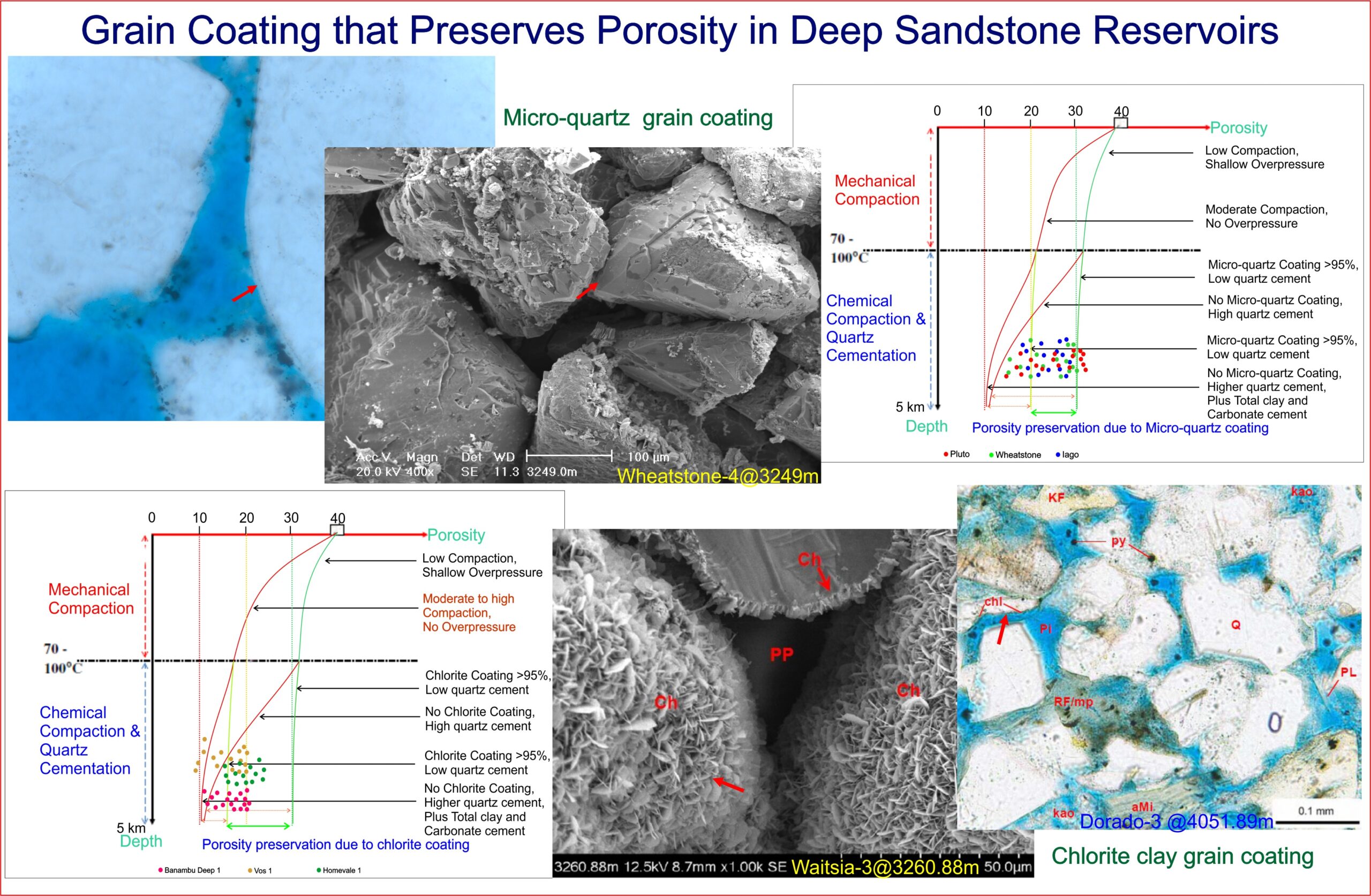The image is an educational infographic prominently titled "Grain Coating that Preserves Porosity in Deep Sandstone Reservoirs" in blue letters on a white background. At the upper left, there is a visually striking picture depicting what appears to be large white objects resembling icebergs against a deep blue center. Central to the infographic, a green heading reads "Micro-Quartz Grain Coating," accompanied by images of gray, porous rocks. To the right of this, a chart illustrates processes like mechanical and chemical compaction. The lower section of the infographic is partitioned into two corners: on the lower right, more detailed images show a closer view of the white objects and blue areas, alongside additional rock samples; on the lower left, another chart mirrors the one seen in the upper right, enhancing the explanation of the grain coating process. The infographic is richly colored with light blue, blue, red, green, gray, black, and purple hues, with the elements somewhat overlapping, contributing to a visually dense but informative layout aimed at educating viewers on the preservation of porosity in sandstone reservoirs through micro-quartz grain coatings.